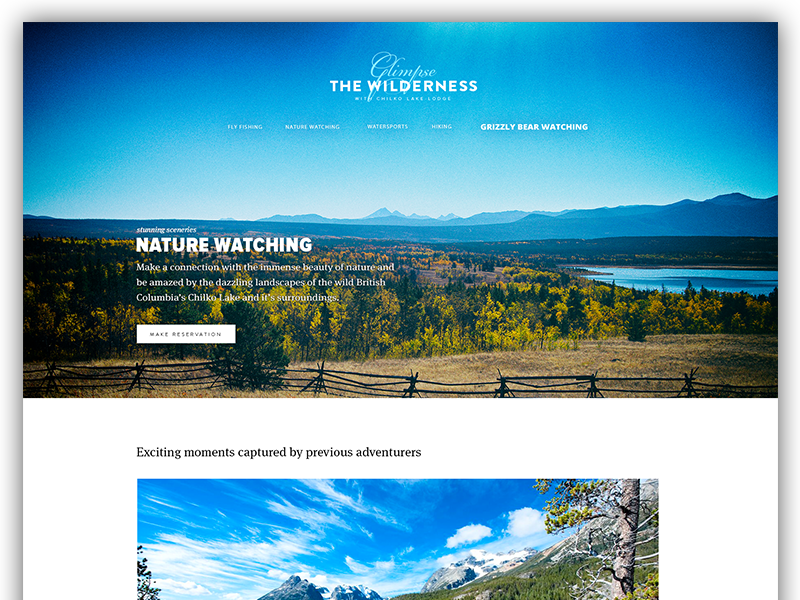**Descriptive Caption:**

On the website "Glimpse the Wilderness," visitors are welcomed with an immersive visual experience of the Chicco Lake Resort, Light Lodge. The central theme of the page is dominated by the bold, large text "Wilderness," though the fine print underneath is difficult to decipher due to the low resolution. Beneath this heading is the navigation bar listing activities: fly fishing, nature watching, water sports, hiking, and prominently, grizzly bear watching, which stands out more than the other links.

The backdrop of the website features a stunning photograph that anchors the aesthetic. The viewer is greeted by a vast grassy field bordered by a rustic, roughly made fence. To the right, a serene lake sparkles, framed by trees that are turning golden, hinting at the arrival of fall. Beyond the lake, majestic mountains rise, shrouded in the soft glow of the horizon. The expansive sky, a clear blue devoid of clouds, stretches endlessly above.

On the left side of the image, promotional text reads: "Stunning scenery, nature watching. Make a connection with the immense beauty of nature and be amazed by the dazzling landscape of the wild British Columbian Chilko Lake and its surroundings." Below this, a prominent white button invites action with the words "Make a Reservation" rendered in black text.

At the bottom of the page, partly obscured, is a teaser photo showing just the upper portion of a sky, dotted with clouds, hinting at the promise of more breathtaking vistas captured by past adventurers.